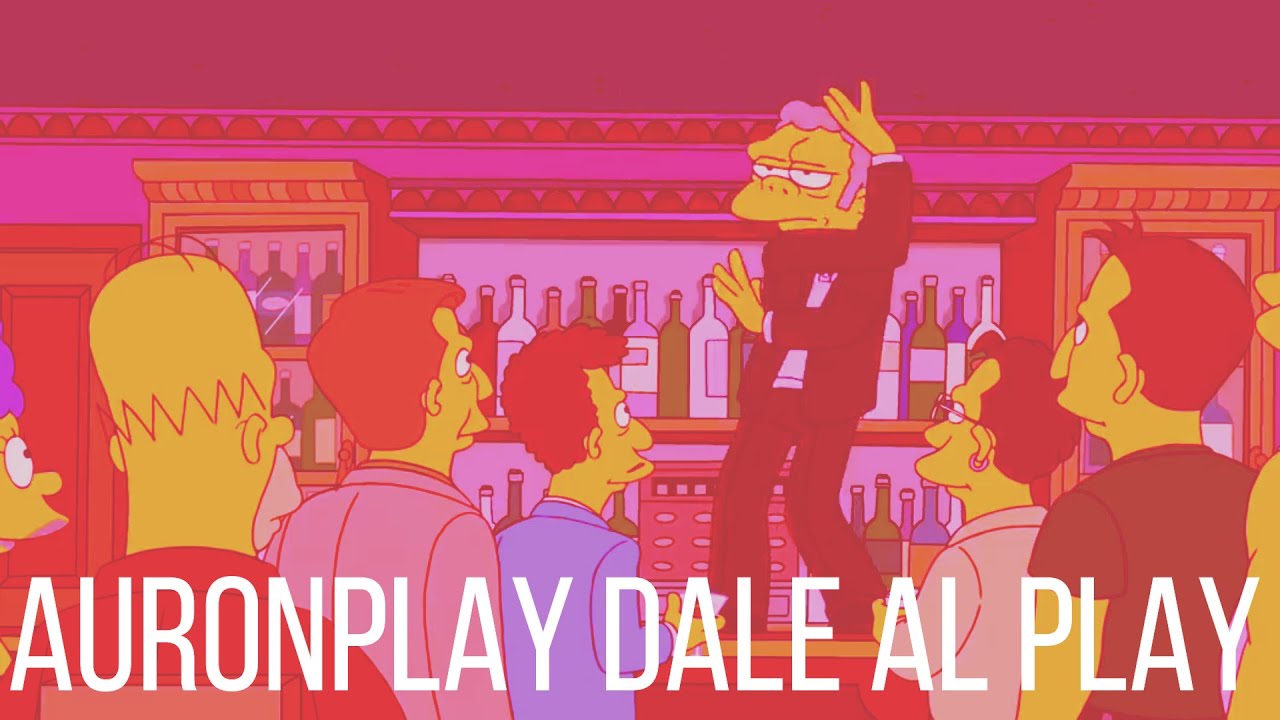This image is a detailed snapshot from the television show, "The Simpsons." The scene unfolds in a bar where a gray-haired bartender, dressed in a black suit with a light-colored shirt, is energetically dancing atop the bar counter. His face exhibits an intense, almost angry expression while his arms are dynamically positioned. Behind him, numerous bottles of various drinks are neatly stacked on shelves along the wall. In the foreground, several patrons, including five other male characters, are captivated by the bartender's performance. On the bottom left, the back of Homer's head is visible as he sits, with Marge standing beside him, her face partially visible with a sprig of her iconic blue hair showing. Spanish text runs across the bottom of the image, reading "A-U-R-O-N-P-L-A-Y-D-A-L-E-A-L-P-L-A-Y."